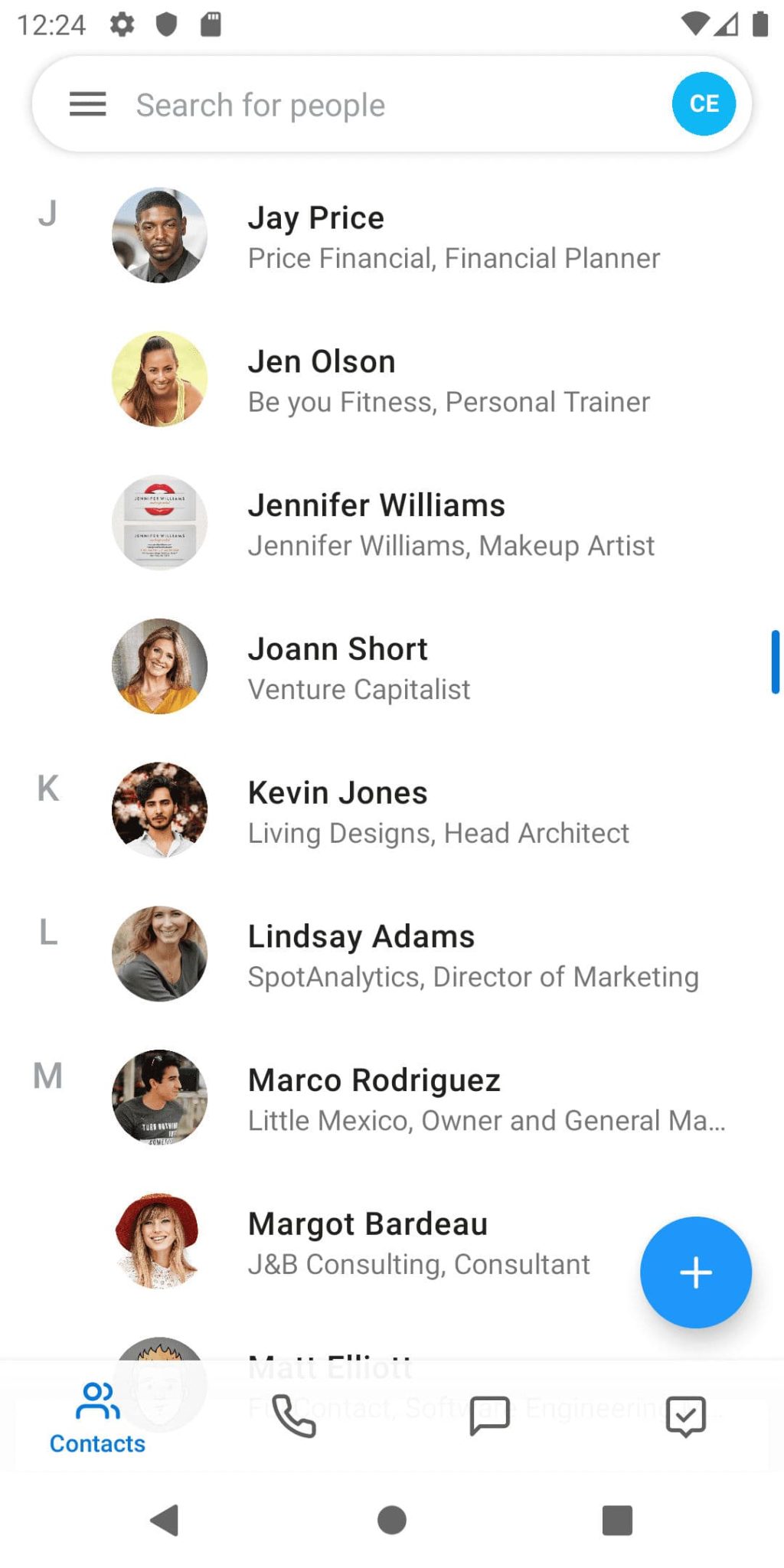Displayed on this smartphone screen is a clean, white background featuring a series of grey icons along the top. On the top left corner, the time reads 12:24, accompanied by icons representing settings, a shield, and an SD card. In the top right corner, grey icons indicate a Wi-Fi connection, cellular signal strength, and a notifications icon. 

Beneath these icons is a search bar labeled "Search for people," flanked on the right by a user profile icon displaying the initials "CE" in white against a blue circular background.

The application lists several individuals, each accompanied by their name, occupation, and relevant professional details. The first person listed is:
- **Jay Price**: Financial Planner at Price Financial
- **Jane Olsen**: Personal Trainer at Be Your Fitness
- **Jennifer Williams**: Makeup Artist
- **Joan Short**: Venture Capitalist
- **Kevin Jones**: Head Architect at Living Design
- **Lindsay Adams**: Director of Marketing at Post Analytics
- **Marco Rodriguez**: Owner of Little Mexico
- **Margot Badeau**: Consultant at J&B Consulting

At the bottom of the screen, there's a row of four buttons: Contacts, Call, Message, and a Check sign. The 'Contacts' button is highlighted in blue, indicating it is currently selected.